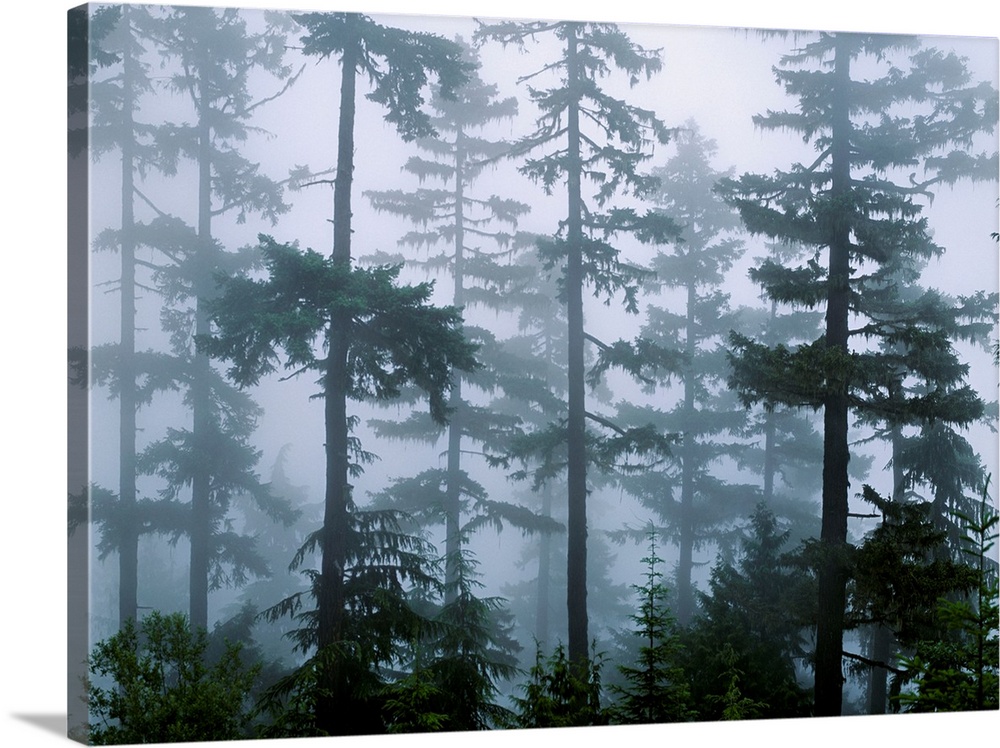This is a photograph of a piece of wall art, printed on a 3D canvas that wraps around the edges for added depth. The image depicts a foggy forest scene with very tall, slender trees featuring narrow trunks and sparse branches. Some trees are visible in the foreground, while others fade into the hazy, light gray background. The trees, characterized by their bare spots and thin limbs with small clusters of leaves, create a sense of depth and mystery. The overall atmosphere is dark and dreary, yet there are hints of darker, vibrant green tones in the foliage. The canvas sits on the ground, slightly turned diagonally, allowing us to see its shadow and enhancing the three-dimensional effect.